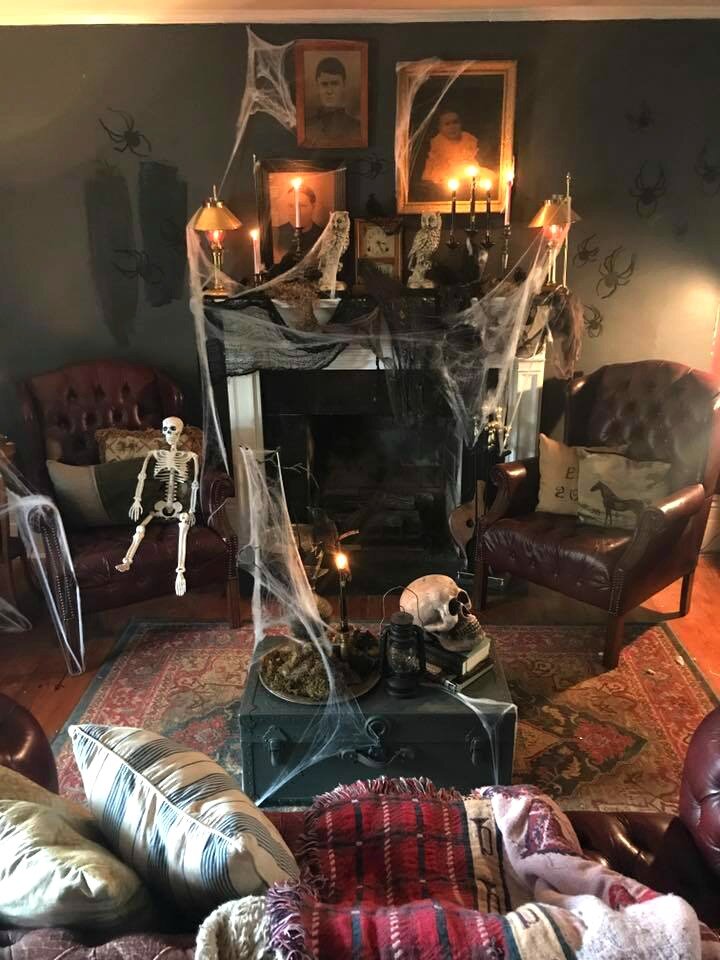The image depicts a cozy living room meticulously decorated for Halloween, captured from a perspective behind a large brown leather couch adorned with pillows on the left and a blanket draped in the middle. Dominating the scene is a gray wall with a central fireplace. The fireplace mantel is festooned with black and gray creepy cloth and an abundance of dangling spiderwebs. Atop the mantel are old black-and-white photographs enveloped in cobwebs, flanked by statues of owls, a central clock, and surrounding candles. On either side of the fireplace, black spiders appear to crawl up the wall, enhancing the eerie atmosphere.

To the left of the fireplace, an old brown leather chair is home to a white skeleton, further draped in cobwebs. Opposite, on the right, another chair features decorative pillows, with one showcasing a horse motif. Centered in front of the fireplace is a vintage black chest, serving as a coffee table, topped with a skull, a book, and an old metal lantern. The entire tabletop and its items are also shrouded in spiderwebs. The scene is completed with a rug beneath the chest, unifying the spooky elements into a single, detailed Halloween tableau.